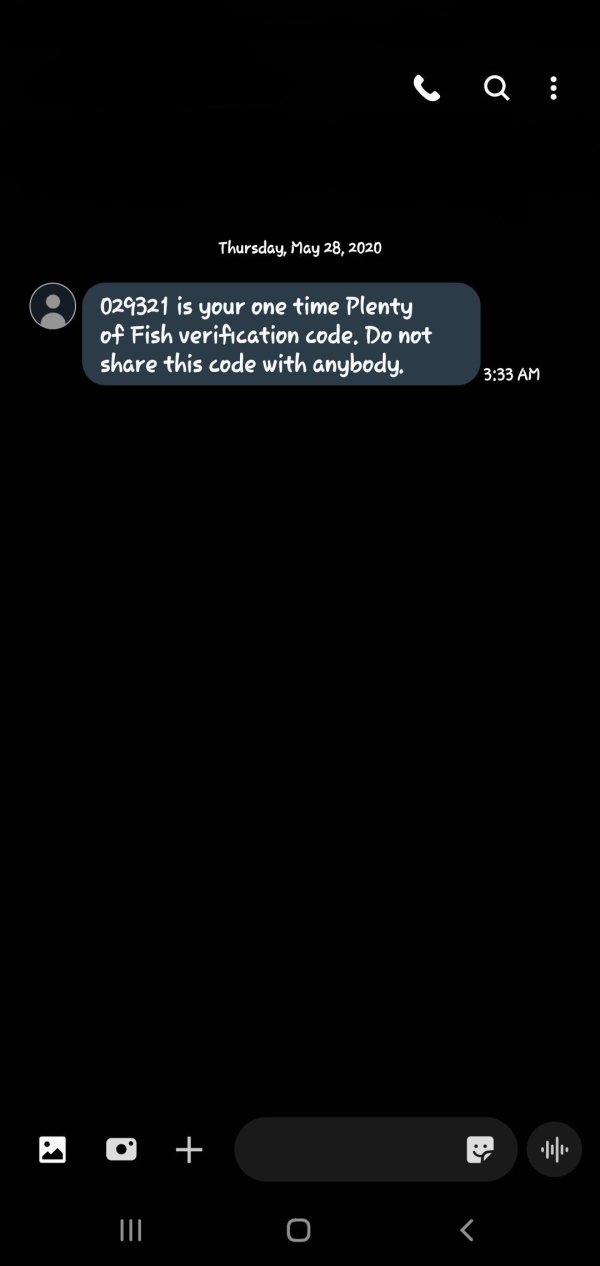**Screenshot Description:**

The screenshot displays a black background indicating a phone's screen. 

**Top Section:**
- In the upper right-hand corner, three icons are visible:
  1. A white phone icon.
  2. A white magnifying glass icon.
  3. Three white vertical dots.

**Upper Center Section:**
- A white timestamp reads, "Thursday, May 28th, 2020."

**User's Avatar and Message Details:**
- Below the timestamp, there is a gray circle with a white outline, featuring a gray silhouette of a person, serving as the avatar for the individual who sent the text.
- The message is contained within a gray box with white text, stating: "029321 is your one-time Plenty of Fish verification code. Do not share this code with anybody." Notably, the words "Plenty" and "Fish" are capitalized.
- The time the message was sent is indicated as "3:33 AM."

**Bottom Section:**
- Towards the bottom, there are several icons and options aligned horizontally:
  - A picture icon depicted in gray with a mountain and possibly a sun.
  - A camera icon.
  - A plus (+) icon.
  - A message bar for entering text with an icon of a piece of paper, characterized by a bent bottom right corner and a smiling face with two eyes.
  - A black circle with white horizontal lines designed for voice recording.
- At the very bottom left, three vertical lines are positioned in a row.
- The center icon is a square with a white border.
- The final icon on the right is an arrow pointing to the left.